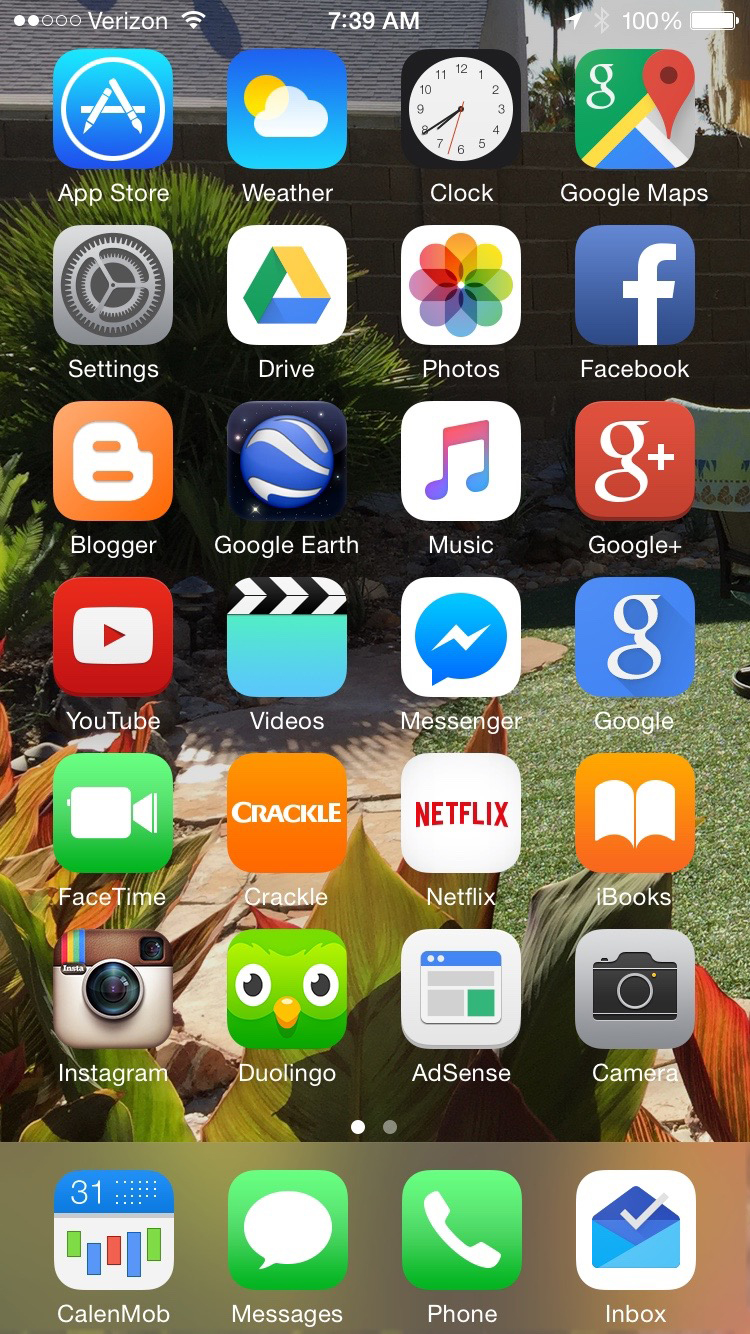In this image, taken against an outdoor backdrop of lush plants and a cozy patio area, the screen of a smartphone is prominently displayed. In the upper left corner, the status bar showcases two out of five signal bars for Verizon, a lit Wi-Fi icon, and the current time, which is 7:39 a.m. The upper right corner displays a full battery icon with a 100% charge.

The smartphone screen features an array of apps organized neatly in rows. The first row from left to right includes the App Store, Weather, Clock (showing 7:40), and Google Maps. The second row contains Settings, Google Drive, Photos, and Facebook. The third row is comprised of Blogger (an orange box with a white "B"), Google Earth, Music, and Google Plus. The fourth row features YouTube, Videos, Messenger, and Google. Finally, the bottom row visible in the image includes FaceTime, Crackle, Netflix, and iBooks.

This meticulous arrangement of apps overlaid on an idyllic outdoor setting creates a juxtaposition between digital and natural worlds.